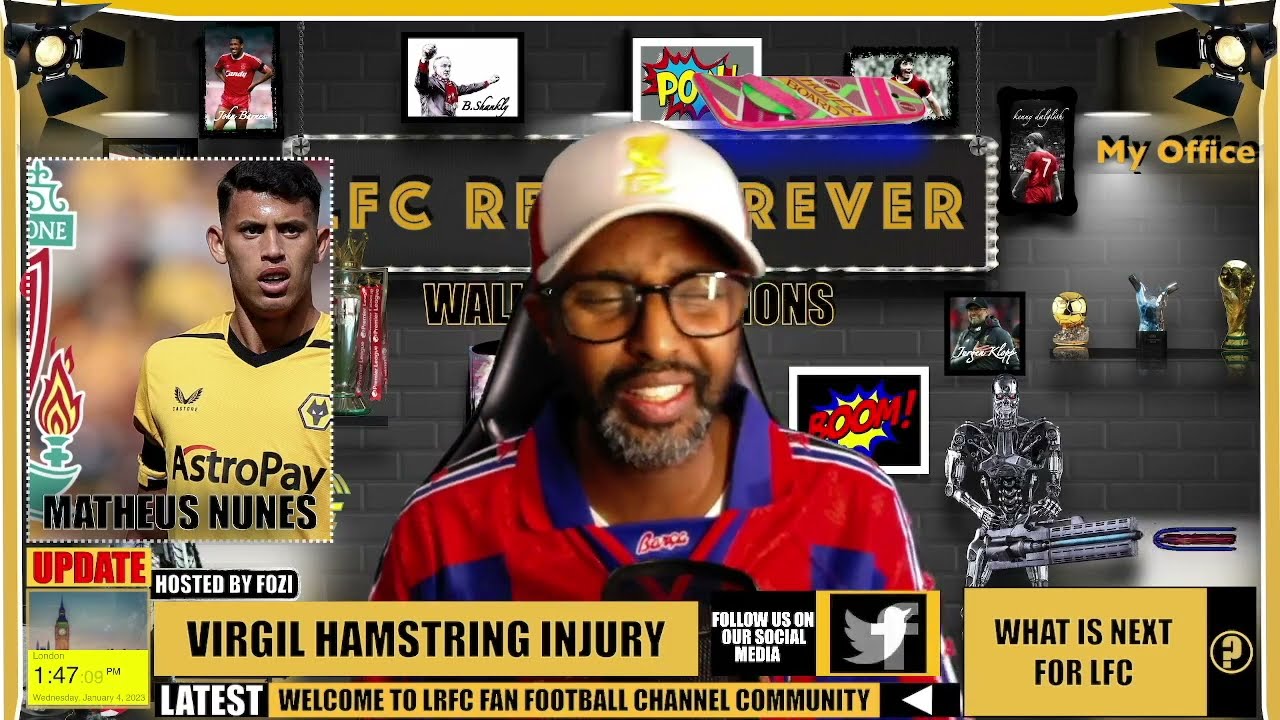The image captures a lively and colorful scene centered around a man of darker skin complexion who appears to be speaking or perhaps in mid-sentence. He is prominently featured, wearing a red shirt with blue and white stripes on the shoulders, a white baseball cap adorned with a yellow emblem, and circular black glasses that complement his gray beard and goatee. His facial expression suggests a smile, with squinted eyes enhancing his engaging demeanor.

To his left, a smaller inset image displays a man in a yellow shirt, identified as Matthias Nunes, presumably a soccer player, with the text "AstroPay" nearby. The image is filled with textual information, including captions such as "Virgil hamstring injury," "latest welcome to LRFC fan football channel community," and "what is next for LFC."

The background is vibrant, featuring a gray brick wall adorned with various pictures, including sports images and cartoon-style graphics with words like "BOOM" and "POW." On the right side of the image, there are several items resembling awards or trophies, adding to the atmosphere of achievement and sports enthusiasm. Additionally, a number "147" is visible on a yellow background in the upper left corner, further enriching the visual detail of the scene.